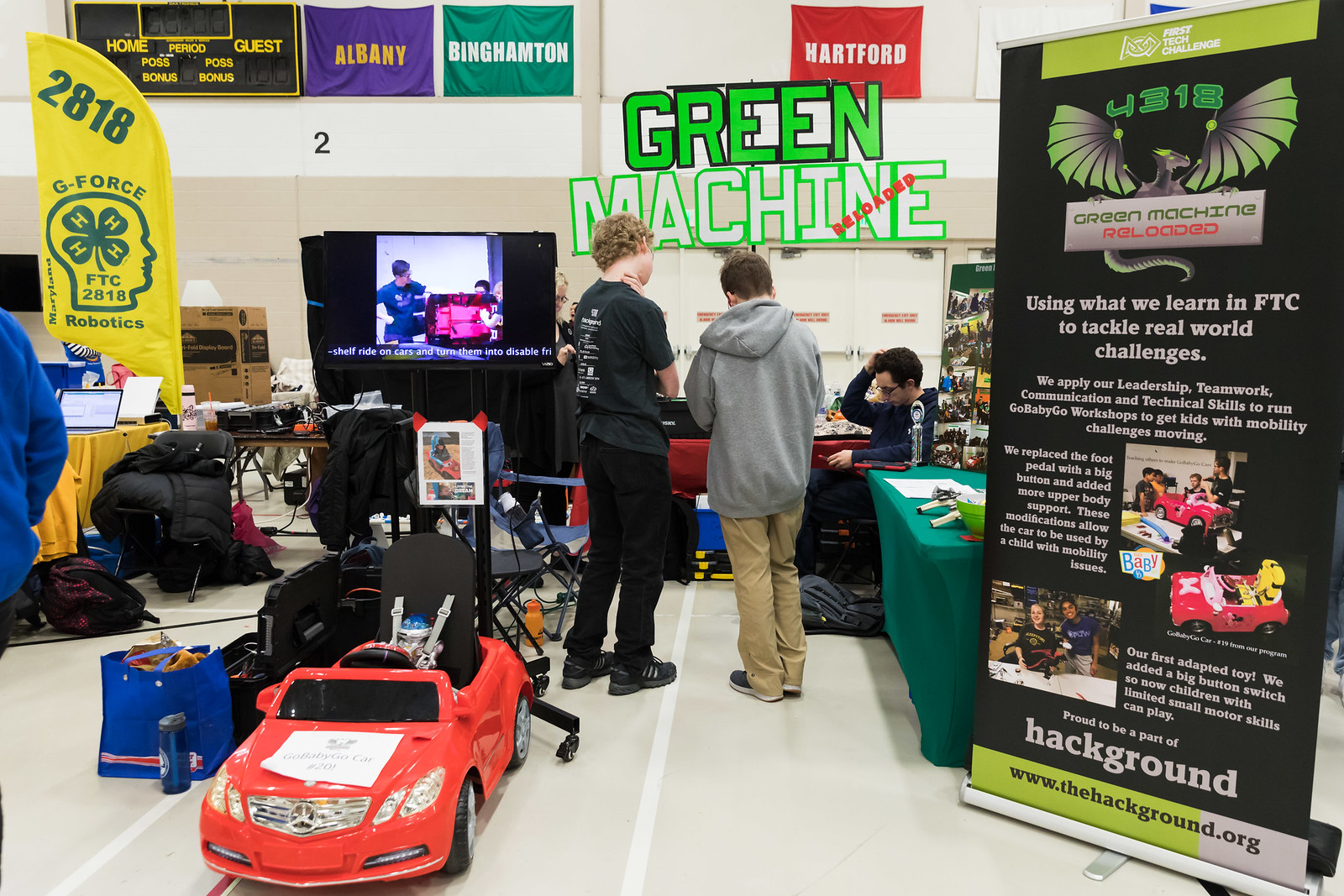The image depicts a small convention, likely held in a gymnasium, featuring two boys standing in the center amidst various banners and displays. The boy on the left, who has blonde hair, is dressed in all black, while the boy on the right wears a gray hooded sweatshirt with beige pants. Prominent in the background is a large banner on the right that states, "Using what we learn in FTC to tackle real world challenges," with additional text detailing their activities. Above the boys, an overlay reads "Green Machine Reloaded," and to the left, there is a small red toy car. The gymnasium has a typical gray floor and multiple people present, including someone seated in a blue hoodie. Additional banners and flags are visible, including a purple banner marked "Albany," and red and green ones labeled "Hartford." There's a black and yellow scoreboard, and a flag displaying "GeForce FTC Robotics." Various items are scattered around, including a blue bag, a blue lamp, and a canteen. The overall atmosphere suggests a children's workshop or a 4-H club event focused on robotics and mobility solutions for kids.